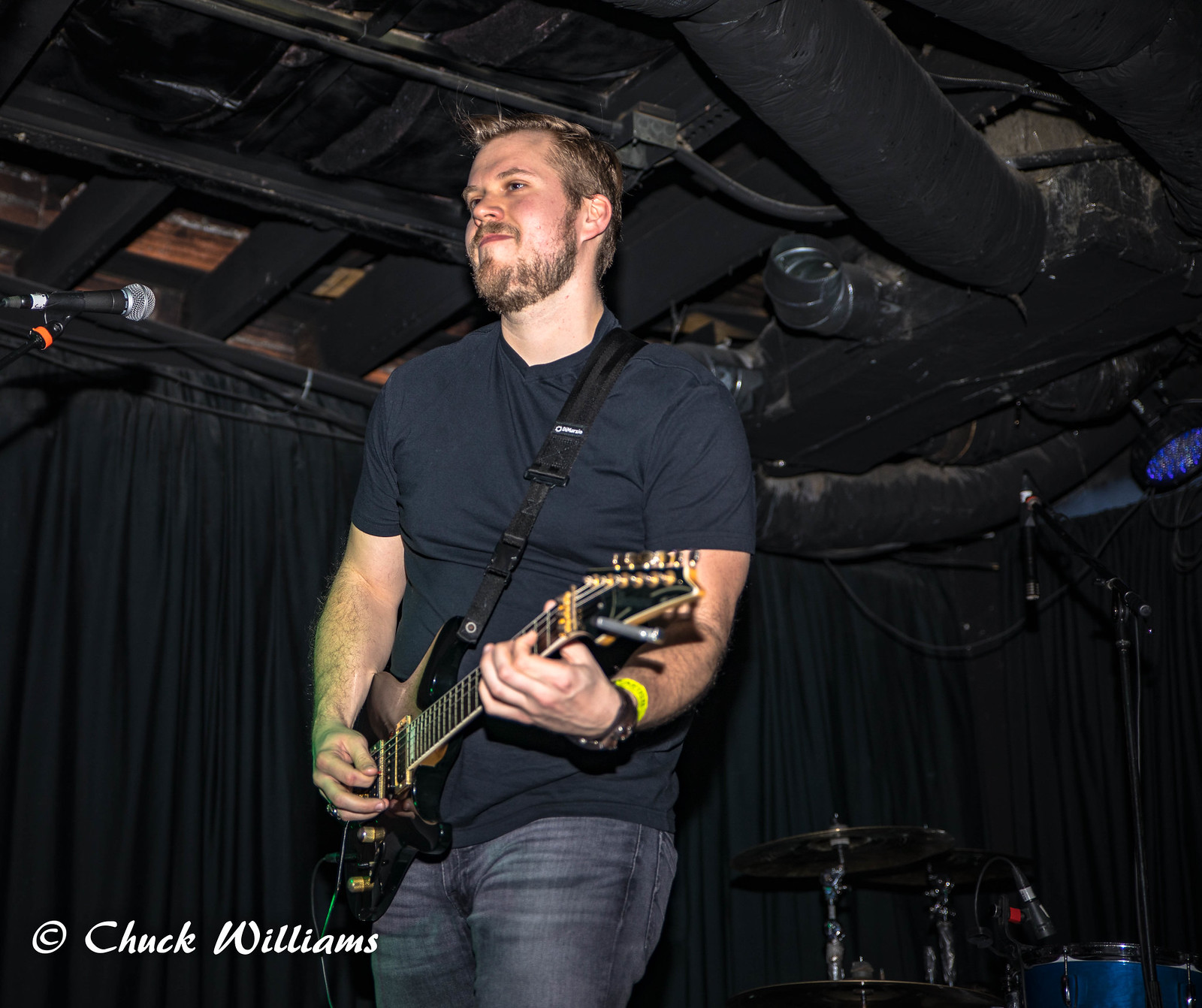The photograph depicts a man in a nightclub or bar setting, performing on a small stage. The man, who has a beard and short cropped blonde hair, wears a black short-sleeved shirt and dark black denim jeans. A watch and bracelet decorate his left hand while he handles a black Stratocaster-type electric guitar adorned with gold fretwork and tuners. The guitar is supported by a nylon strap slung over his left shoulder. 

The man stands with his body facing towards the bottom left corner and his face turned towards the top left corner, looking out into the crowd. A microphone stand is positioned in front of him, although he is not singing. Behind him, there is a drum kit that appears unmanned, featuring blue drums with gold and bronze cymbals, all properly mic'd. A heavily pleated black fabric curtain forms the backdrop of the stage. The stage ceiling, visible above him, displays rafters and various silver vent pipes.

In the bottom left corner of the photograph, the white text reads "Copyright Chuck Williams."